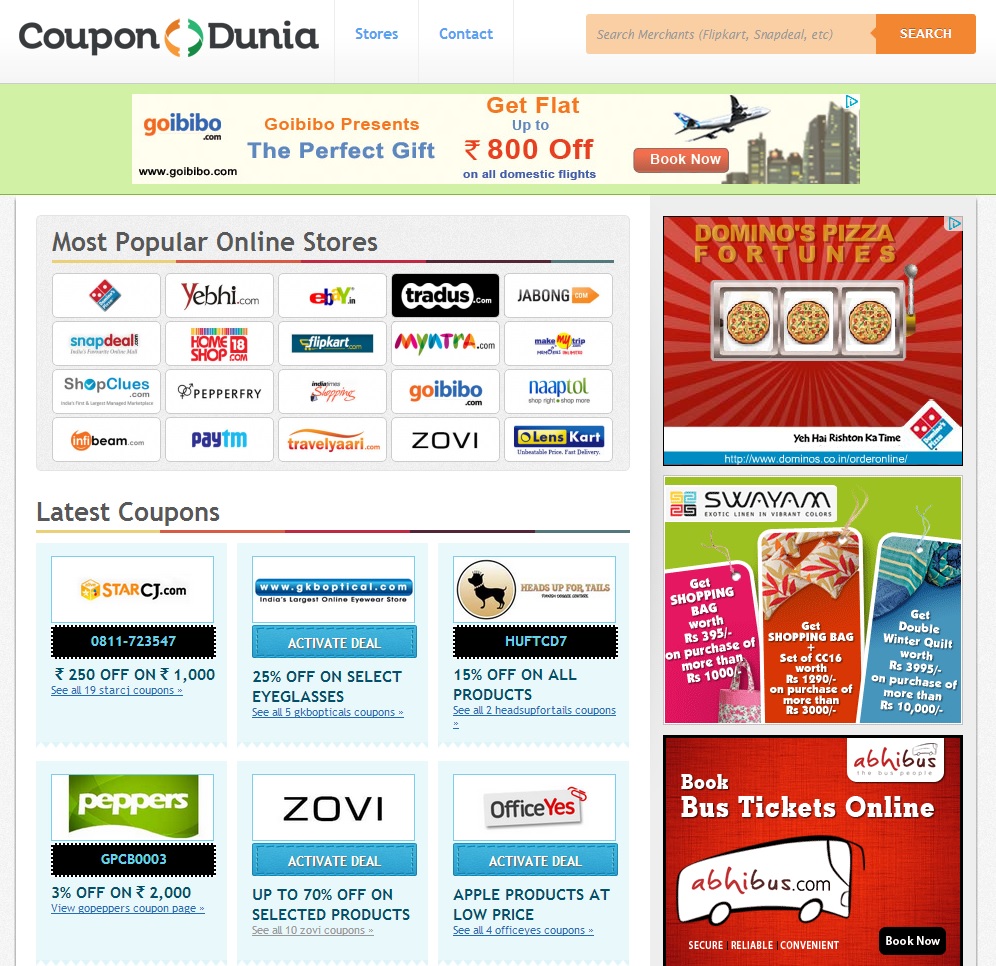Screenshot Description:

The screenshot features a website interface filled with various banners, bars, and advertisements. 

1. **Header Section:**
   - *Coupon Dunia Logo:* Positioned on the upper left-hand side, displaying in an orange-to-green gradient with the logo in between the words "Coupon" and "Dunia".
   - *Navigation Links:* Includes "Stores" and "Contact" in blue font next to the logo.
   - *Search Bar:* Available for searching merchants like Flipkart, Snapdeal, etc. The search bar is light orange, with the text "search" in white font.

2. **Promotional Banner:**
   - *Title:* "Go eBeebo presents the perfect gift".
   - *Offer Details:* "Get flat up to 800 off" in bold text with "800 off" in red and "Get flat" in orange. "Perfect gift" is highlighted in blue.
   - *Subtext:* "On all domestic flights" written under the "800 off" text.
   - *Call-to-Action Button:* A "book now" button paired with an airplane graphic flying towards some buildings.

3. **Popular Stores Section:**
   - *Heading:* "Most popular online stores".
   - *Store Logos:* Displays miniature banners/buttons for various online stores such as Yebhee.com, Pepperfry, Paytm, eBay, Zovee, and others.

4. **Latest Coupons:**
   - *Heading:* "Latest coupons".
   - *Details:* Showcases six coupons available for different sites, each offering a certain percentage off.

5. **Advertisements:**
   - *Domino's Pizza:* Features a slot machine graphic with three pizzas and the Domino’s logo on the right-hand side.
   - *Swayham Ad:* Depicts home goods with three tagged items, presumably with some text details about the products.
   - *Abhebus Ad:* Displays the Abhebus logo to the right and highlights "Book Bus Tickets Online" using a graphic of a bus. The URL "Abhebus.com" is in red text. Below it, the text states "Secure, Reliable, Convenient" on a red background accompanied by a black "Book Now" button in white font.

This detailed description provides a comprehensive understanding of the website's visual elements and the functionality presented in the screenshot.